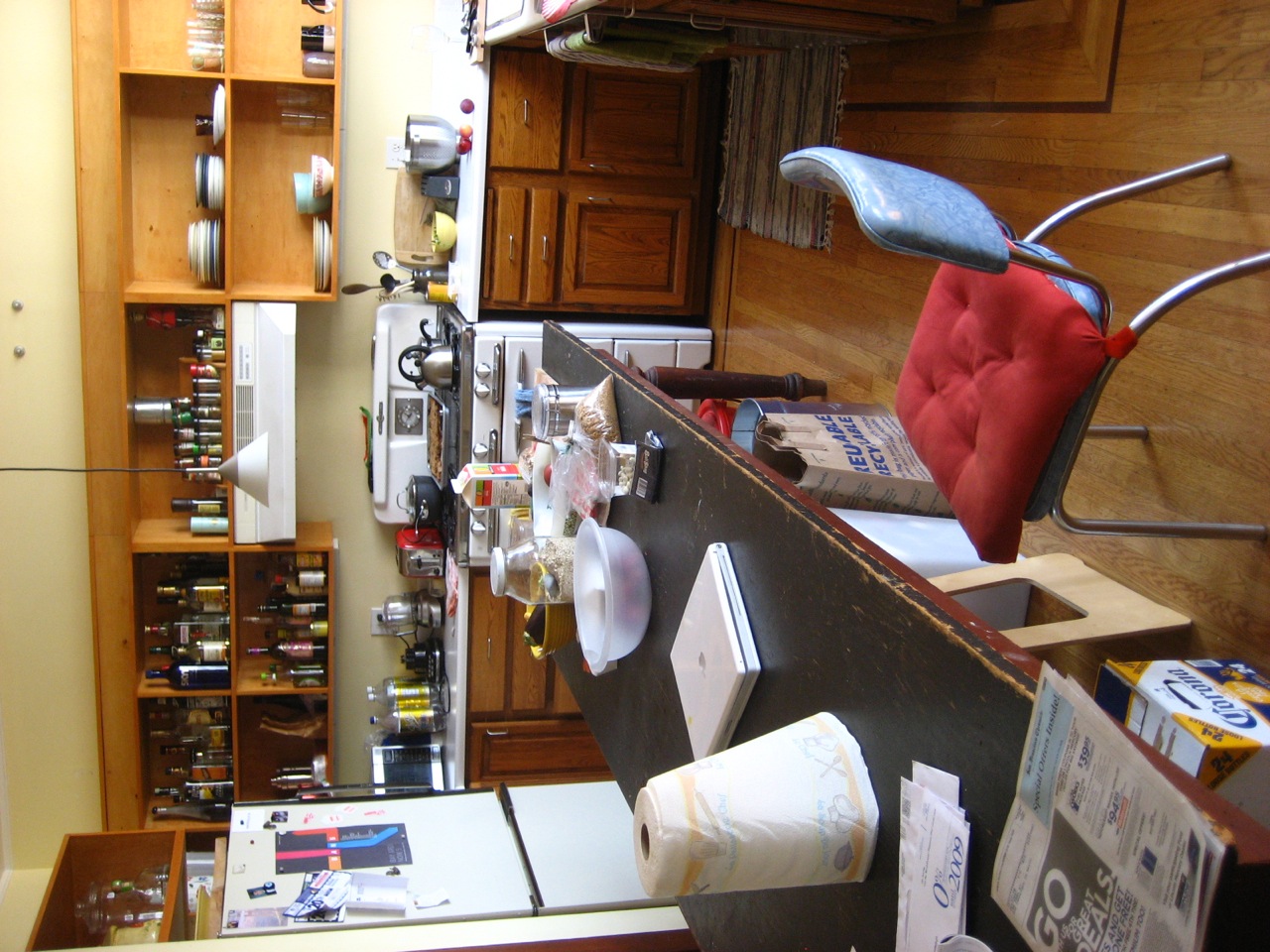This image depicts a bustling kitchen scene centered around a long, dark brown table with red trim along its bottom edge and brown legs. On the table lies a newspaper prominently featuring the word "GO" alongside some enticing deals, flanked by a roll of paper towels decorated with yellow and blue designs, standing upright. A variety of items like a plastic bowl, juice boxes, and food jars clutter the surface. Beneath the table, bags and a box of Corona beer in white and blue add to the organized chaos.

A light blue chair with a sturdy back and silver legs stands out with its orange-red pillow. Brown oak cabinets line the walls, hosting an array of tall jars, bottles, seasoning containers, blue and white plates, and cups. A computer sits on the countertop amidst this culinary landscape. 

The refrigerator, adorned with magnets and photos, stands sentinel while a white stove, crowned with a silvery tea kettle, boasts a microwave and a pan containing food. Near the stove, a mixing bowl and a jar with a spatula provide evidence of recent cooking. The sink area includes a dish towel hanging over a rack, contributing to the lived-in feel of the space.